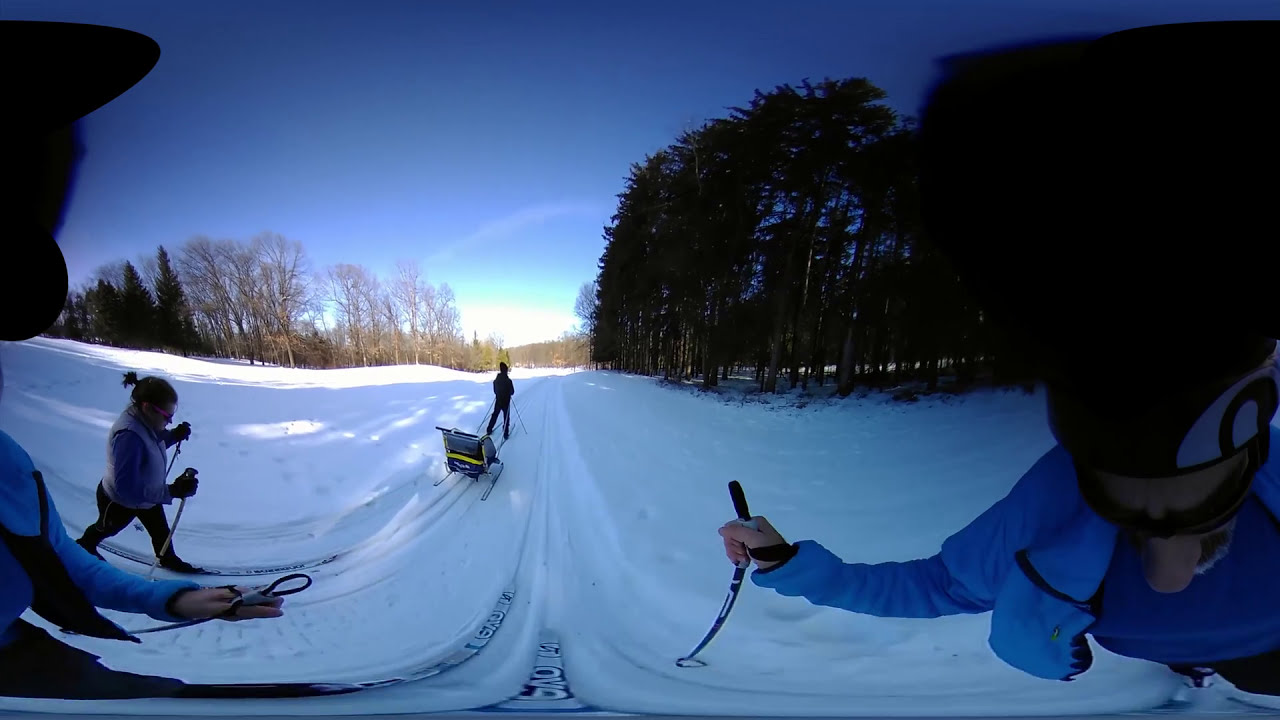The image displays a 360-degree panoramic view from an action cam mounted on a helmet, atop a snow-covered trail set for cross-country skiing. The central figure, wearing a blue jacket, blue shirt, black pants, and a black helmet, is holding ski poles. This helmet-mounted perspective slightly distorts the view of the person. 

To the left, a woman dressed in a blue or purple coat and black pants is also skiing, while in front, a man in all black attire and a black skullcap pulls a gray, blue, and yellow sleigh that might be carrying a child. The trail appears between two types of trees: leafless ones on the left and green pine trees with brown stems on the right. A building with visible windows peeks through the trees on the right.

The white snow is thick, and ski tracks create two distinct paths that diverge into the distance. The bright blue sky with sporadic white clouds overhead adds to the clear, crisp winter day ambiance, perfect for this cross-country skiing adventure.